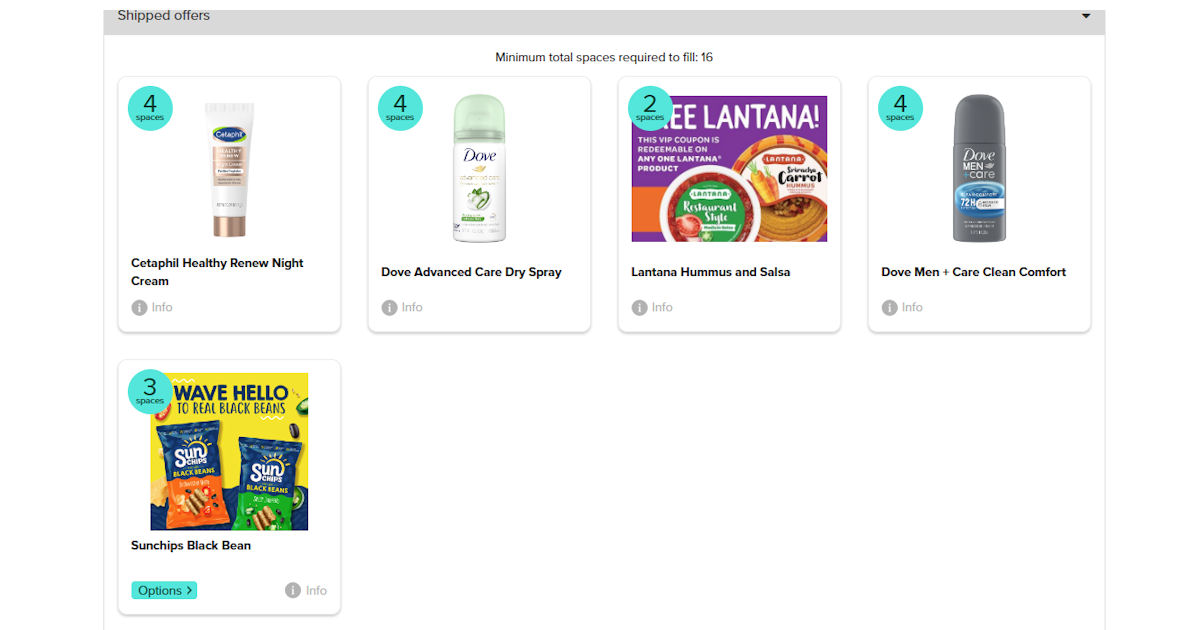The image is a screenshot from a website displaying a section titled "Shipped Offers." At the top, there's a notice indicating a minimum total requirement of 16 spaces that must be filled. Each corner of the product images shows a teal circle with the corresponding number of spaces each item occupies.

- **Cetaphil Healthy Renew Night Cream**: Allocated 4 spaces, marked in a teal circle.
- **Dove Advanced Care Dry Spray**: Allocated 4 spaces, marked in a teal circle, and positioned to the right of the Cetaphil product.
- **La Tana Hummus and Salsa**: Located to the right of the Dove spray, this product has 2 spaces left, indicated in the corner.
- **Dove Men+Care Clean Comfort**: Positioned next, occupying 4 spaces, as shown in the teal circle.
- **Sun Chips Black Bean (Wave Hello to Real Black Beans)**: The final product listed in this category, with 3 spaces left, indicated in the corner. The image also features bags with green and orange accents. 

The layout emphasizes the products and the remaining spaces required to reach the shipping minimum.